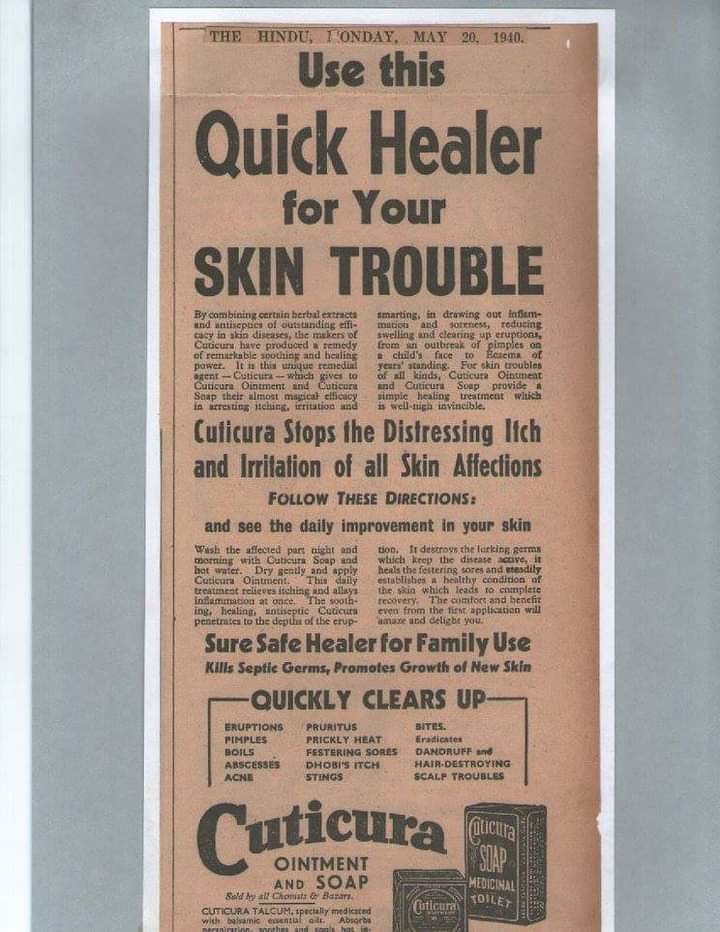The image is of an old, yellowed newspaper advertisement from "The Hindu," dated Monday, May 20th, 1940. The headline reads, "Use this Quick Healer for Your Skin Trouble." The advertisement promotes Cuticura, a remedy for skin afflictions, with large text proclaiming, "Cuticura stops the distressing itch and irritation of all skin affections. Follow these directions and see the daily improvement in your skin." It provides detailed usage instructions: wash the affected part night and morning with Cuticura soap and water, dry gently, and apply the ointment. The advertisement emphasizes that Cuticura is a "sure, safe healer for family use," known for killing septic germs, promoting new skin growth, and quickly clearing up conditions like eruptions, pimples, boils, abscesses, acne, pruritus, prickly heat, festering sores, Dobie's itch, stings, bites, dandruff, and other hair-destroying scalp troubles. The bottom of the ad mentions that Cuticura comprises both ointment and soap, and is sold by chemists and in bazaars. The whole advertisement has a distinctly old look, faded with time, and includes a small, faded black image of the product.